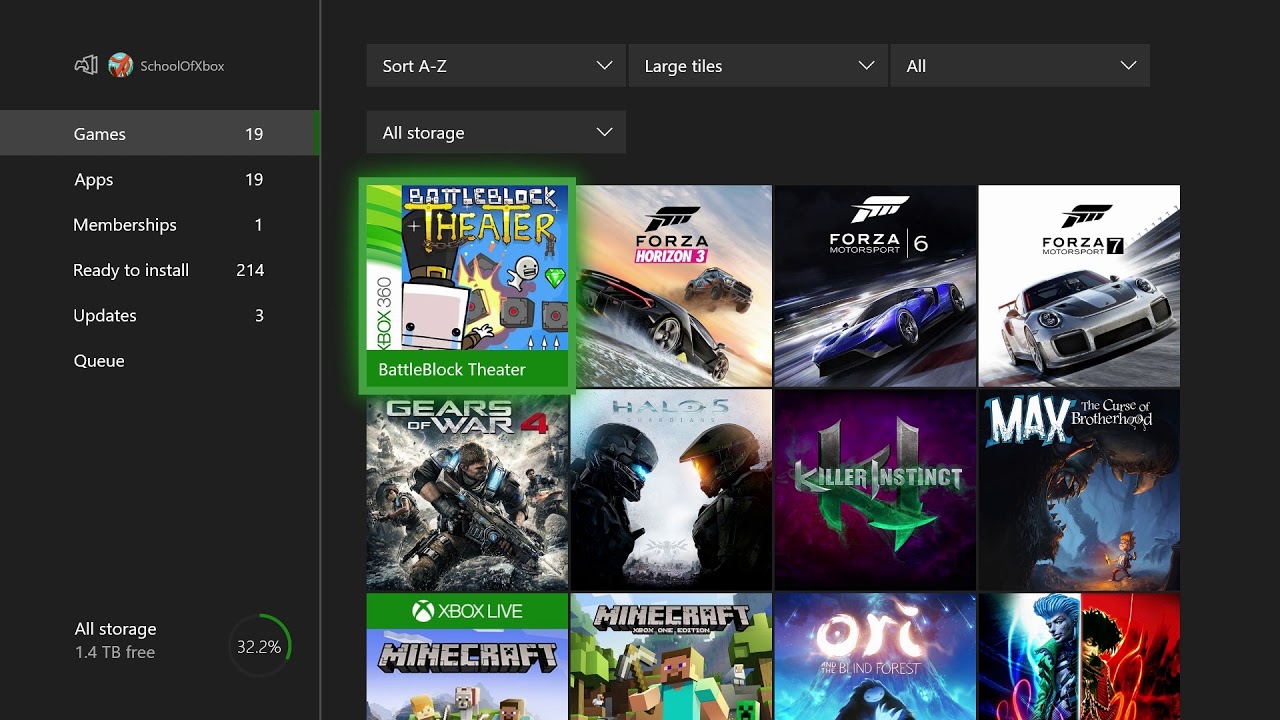In this image set against a solid black background, the upper left corner features the Xbox logo, alongside a circular emblem with an orange character reminiscent of Gumby against a blue backdrop. Just below this, a gray-highlighted section displays the word "Games" followed by the number "19" in white text.

Running down the left side of the image, several categories are listed in white text on a black background: "Apps 19," "Memberships 1," "Ready to install 214," "Updates 3," and "Queue."

To the right of these categories, there is a display of game images sorted alphabetically. The first row includes:
1. "BattleBlock Theater"
2. "Forza Horizon 3"
3. "Forza Motorsport 6"
4. "Forza Motorsport 7"

The second row showcases:
1. "Gears of War 4"
2. "Halo 5: Guardians"
3. "Killer Instinct"
4. "Max: The Curse of Brotherhood"